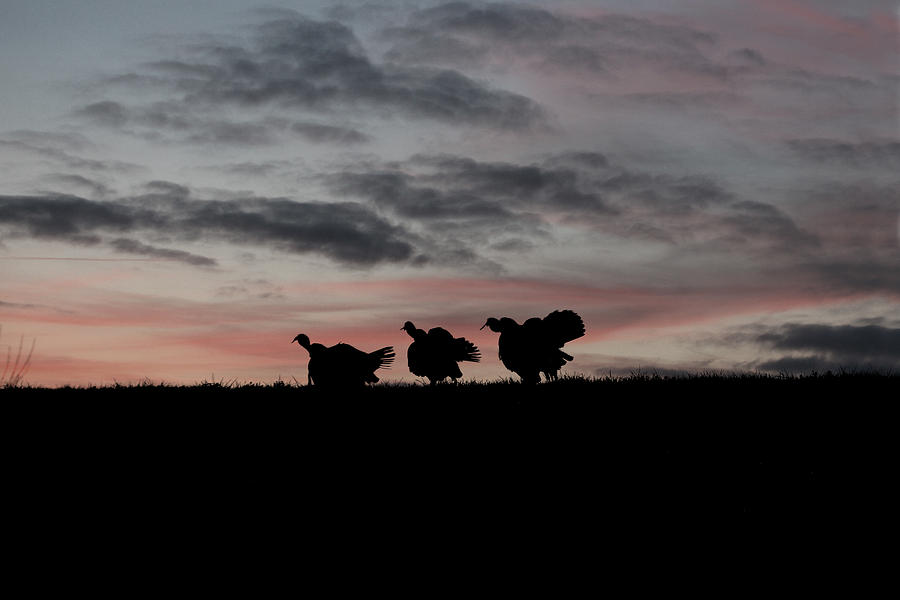In this captivating photograph, the evening sky sets a dramatic backdrop illuminated in hues of pink and light orange, suggesting either dawn or dusk. The sky is adorned with dark gray, wispy clouds that add a sense of depth to the image. Below, a shadowy foreground features a short grass field, so dark it's difficult to discern completely if it's grass or dirt. Along the horizon, which occupies about one-third of the image, three turkeys stand out in sharp silhouette. These turkeys, with their characteristic thicker necks and larger feathers, are perfectly aligned side by side, facing to the left, positioned centrally within the frame. Their dark forms contrast beautifully against the colorful sky, creating a serene yet striking scene reminiscent of rural woodlands or perhaps an Amish countryside at twilight.